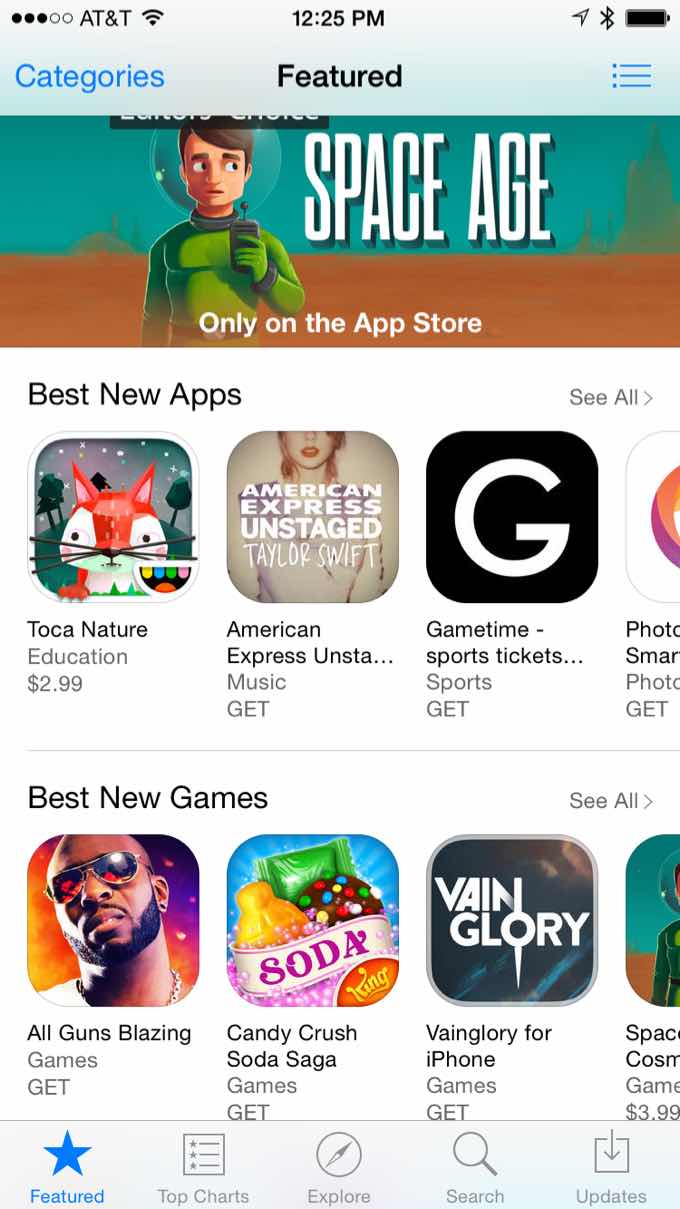This image, taken from an AT&T phone, showcases the featured page of an app store. On the left side, the word “Categories” is prominently displayed in blue letters, while “Featured” is in black. To the right, there are three horizontal lines accompanied by dots, indicating a clickable menu option.

In the upper section of the app store, there is an advertisement featuring a cartoon man holding a walkie-talkie, labeled “Space Age.” The text below reads, “Only on the App Store.” The background features a gradient transition from brown at the bottom to teal at the top, with city buildings faintly visible. The character appears to be an astronaut, identified by the bubble-like helmet around his head.

Scrolling down, the heading “Best New Apps” can be seen. Below this, on the left, is an app titled “TOCA Nature.” Adjacent to it is a promotional image of Taylor Swift, labeled “American Express Unstaged Taylor Swift.” Further down is another app titled “Game Time Sports Tickets,” displayed with a large white “G” on a black background. The text for the subsequent app is partially cut off.

Further down, the section “Best New Games” is visible, featuring “All Guns Blazing,” “Candy Crush Soda Saga,” “Vainglory,” and another game title that is also partially cut off.